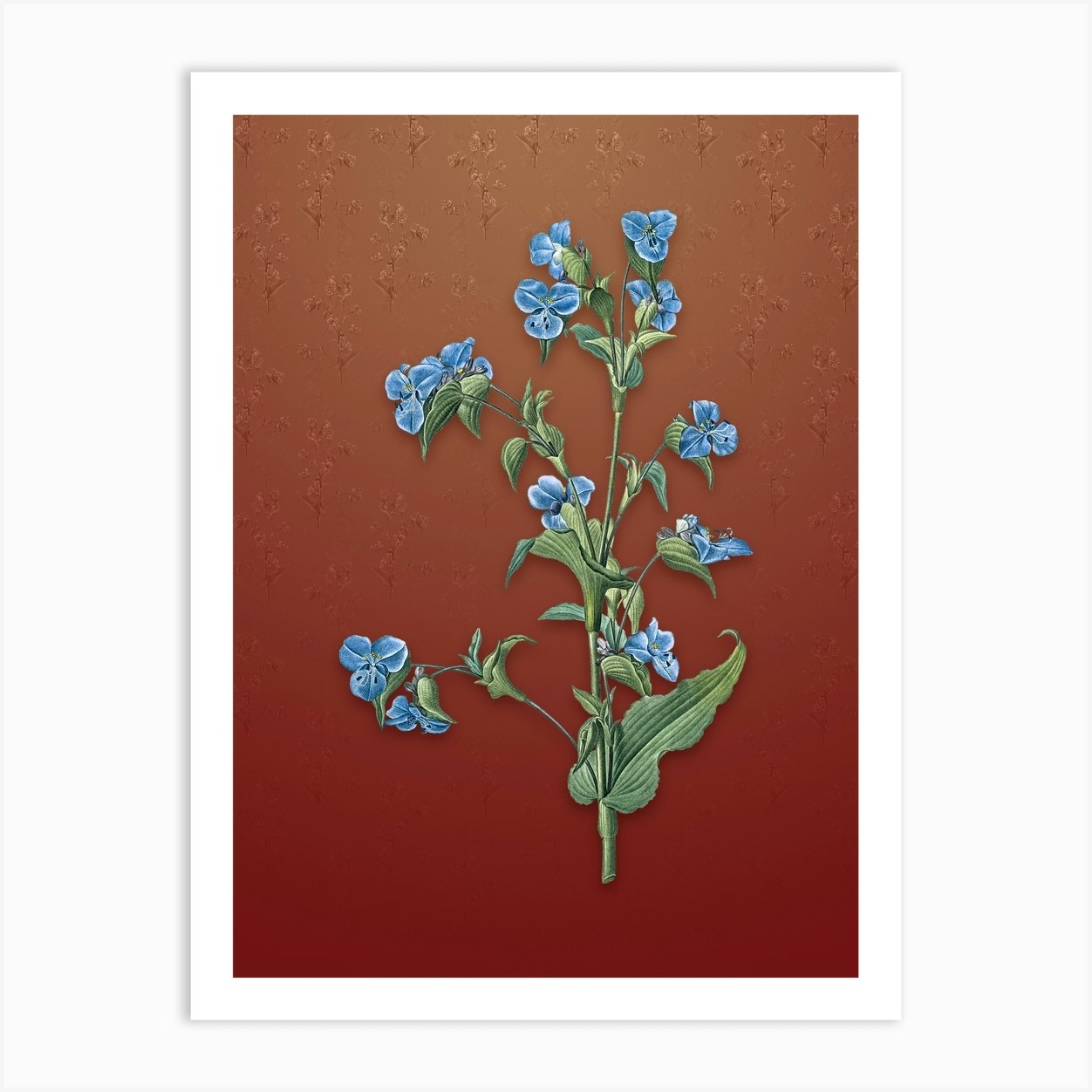This is a detailed, computer-generated, matted art piece featuring an intricate illustration of small blue flowers, possibly violets, with various green leaves and stems. The flowers and leaves are arranged vertically, directly facing the viewer, and the entire composition has a realistic, almost 3D quality. The background of the image transitions from a lighter shade at the top to a deeper brown at the bottom, creating an ombre effect. This brown background is adorned with numerous miniature, repeated patterns of similar flowers, subtly engraved into the surface, giving the image depth. All of this is framed by a white matte, emphasizing the composition. The overall color scheme includes shades of blue, green, brown, and white, creating a harmonious and visually appealing piece. There is no text present on the artwork.